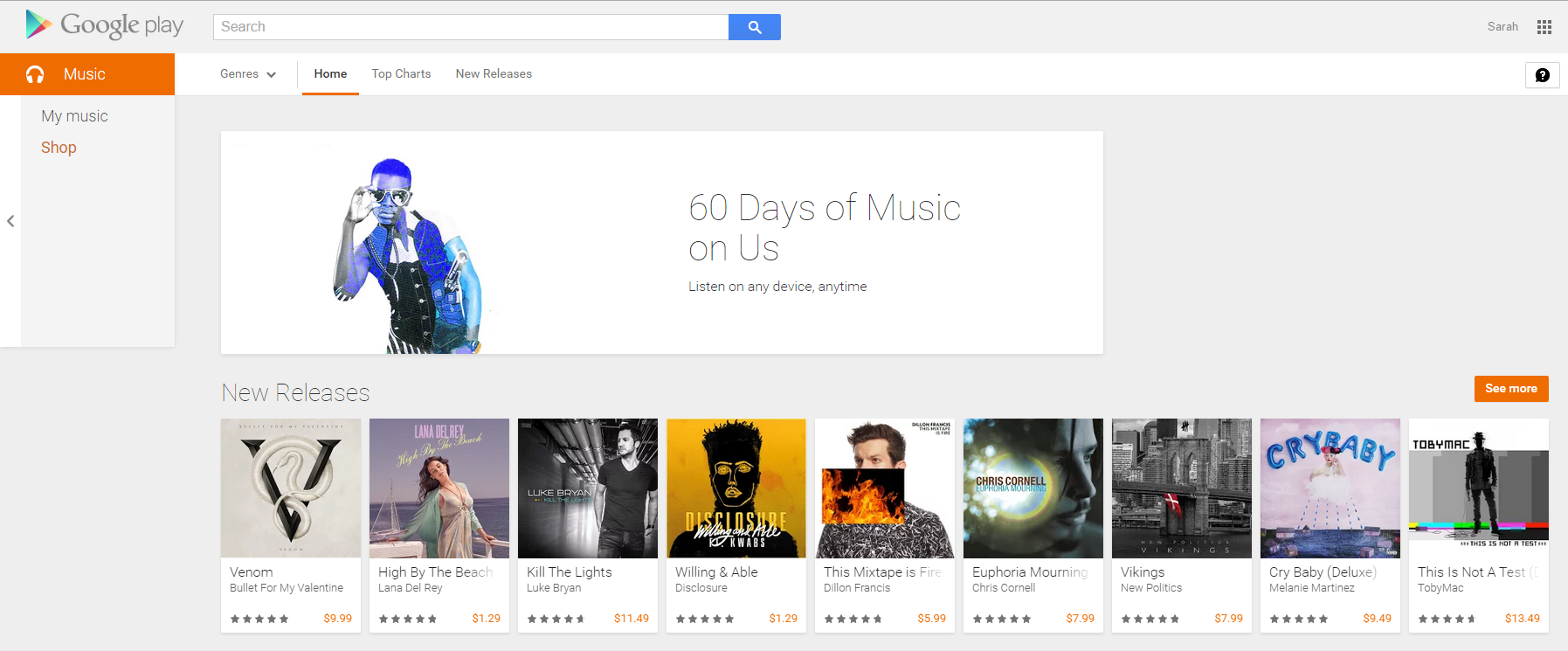This image captures the Google Play Music web page, characterized by its signature green, red, yellow, and blue Google icon. At the top of the page, there is a prominent search bar. Below the search bar, a navigation menu displays options such as "Music," highlighted in an orange bar with white letters and a white headphone icon. Adjacent to "Music," the menu includes links labeled "Genres," "Home," "Your Charts," and "New Releases."

The main section of the page features an advertisement showcasing an African American individual with striking blue hair, wearing striped pants, a leather vest, a white shirt with a blue scarf, all set against a backdrop with a predominant blue tint. The ad promotes "60 Days of Music on Us."

Below the advertisement, the page presents a list of new music releases. "Venom," one of the featured titles, is depicted with a V shape entwined by a snake. Another highlighted release is "Cry Baby."